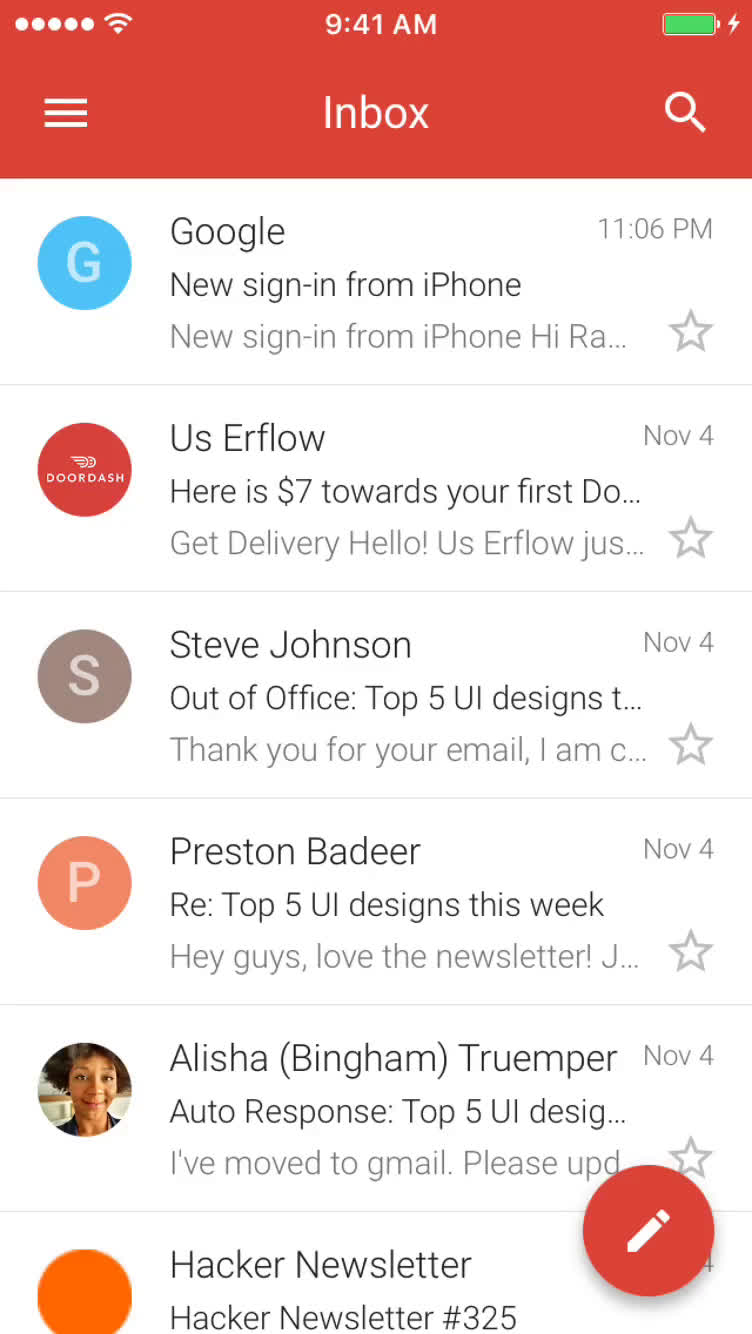Screenshot of a mobile inbox interface, captured at 9:41 AM while the phone is charging, indicated by a full green battery icon in the top-right corner. The top of the screen features an orange banner with four white circular buttons, including a Wi-Fi signal icon in the left corner. Centered on the banner, "Inbox" is displayed in white font, accompanied by three white horizontal lines and a magnifying glass icon.

The inbox displays several emails. The first email, from Google, marked with a blue circular profile icon containing a "G", notifies the user of a new sign-in from an iPhone at 11:06 PM. The subject of the email is "New sign-in from iPhone" and the preview reads "Hi, R.A." with a star icon on the right.

The second email, from DoorDash, is titled "US Airflow, here is $7 towards your door." The preview reads "First DoorDash, get delivery, hello, US Airflow." It was sent on November 4th and also features a star icon.

Further emails include a message from Steve Johnson titled "Out of office, top five UI designs" and additional messages from Preston Badir, Alicia Bingham, and the Hacker Newsletter.